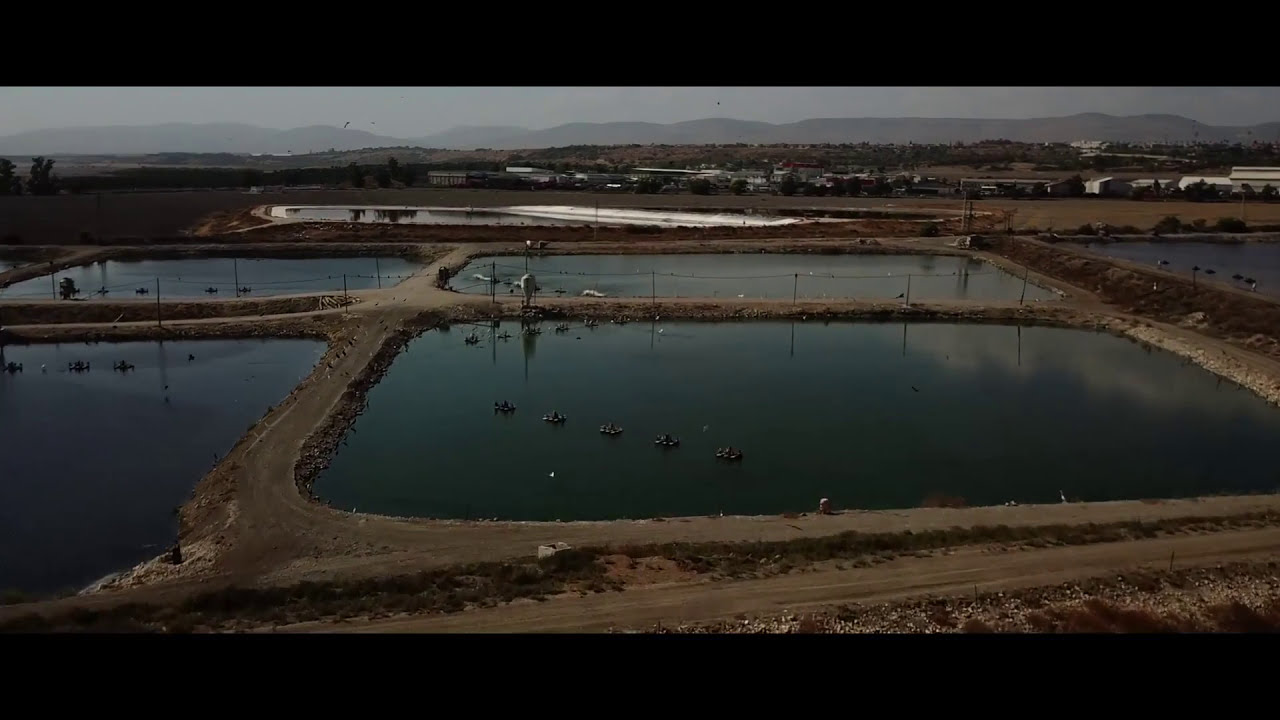The image, captured from a high vantage point, possibly by a drone, depicts a fish hatchery with four prominent rectangular ponds aligned in a square formation. Elevated dirt paths divide and provide access to each pond. Floating buoys, likely indicating netted sections for different fish, are visible atop the water. Extending outward from the ponds are several metal poles and power lines. In the background, partially obscured, is a fifth irregularly-shaped pond. Behind the ponds lies a cluster of short buildings, and further still, a range of mountains. The sky is overcast and gray, casting a foggy, almost smoggy, atmosphere over the scene.